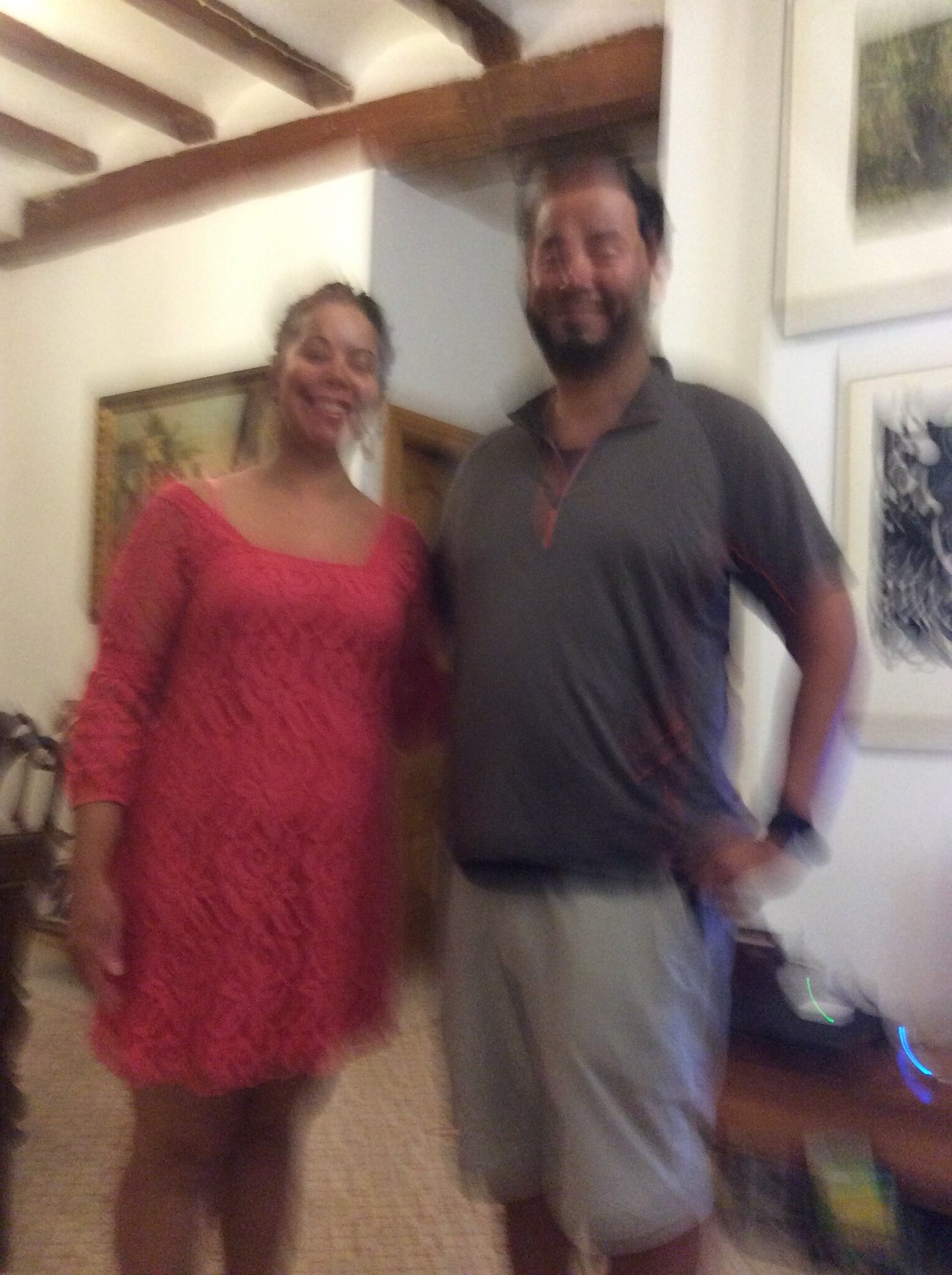In this slightly blurry photograph, two individuals are standing in a well-lit room adorned with artistic paintings. On the left, a woman with a medium-dark skin tone exudes elegance in a knee-length, red lace dress. Her hair is neatly pulled back, revealing her joyful smile. On the right, a man with a similar medium skin tone stands confidently in a gray polo shirt accented with red details near the neckline and a pair of light gray shorts that graze his knees. He wears a black belt and sports a black watch on his right wrist. Despite his closed-mouth smile, his black scruffy beard adds a rugged charm to his appearance. The backdrop features white walls complemented by wooden ceiling details, enhancing the cozy ambiance of the room.